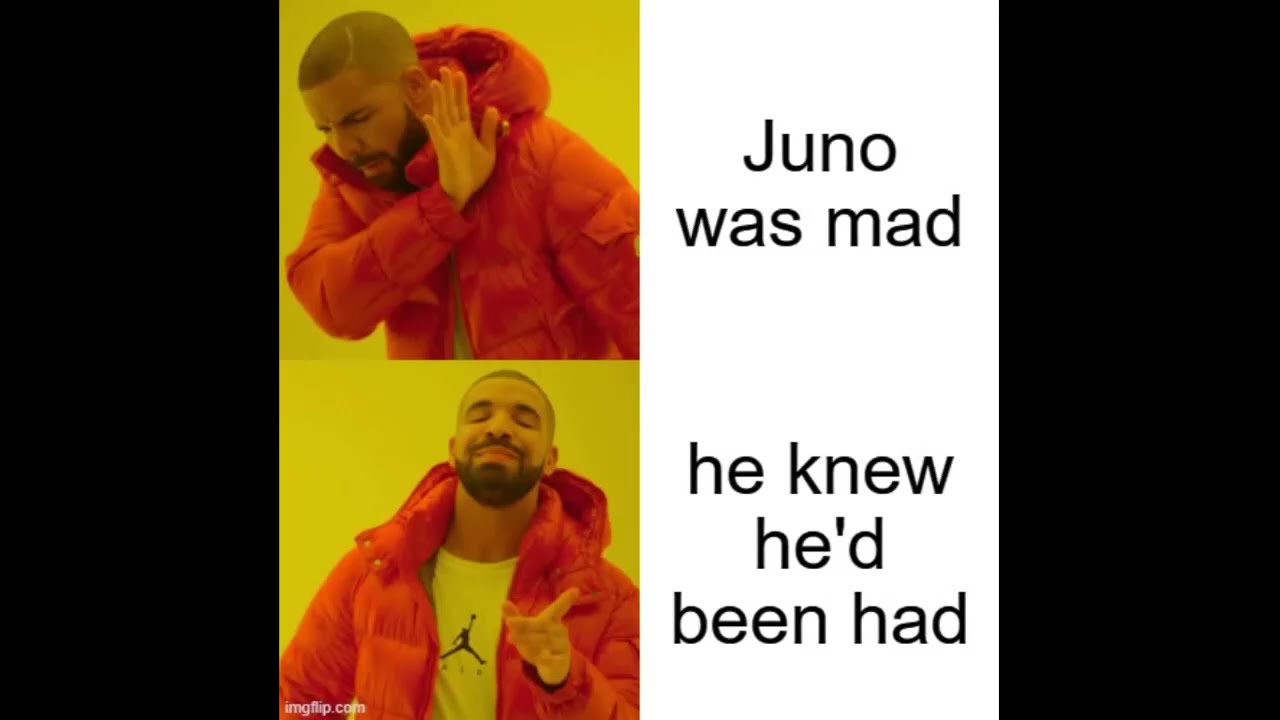The image features a well-known meme format using two frames of the musician Drake, positioned on the left side against a yellow background. Both images of Drake are accompanied by black borders on the left and right of the overall picture, creating a striking contrast. In the top frame, Drake, a black man with black hair styled in a fade and a beard, is seen wearing a puffy red coat. His face is turned to the left with his hand raised, expressing a gesture of disapproval. The text to the right of this image reads, "Juno was mad." In the bottom frame, Drake, now with his coat open to reveal a white t-shirt featuring a black Air Jordan logo, is pointing towards the camera with a confident smirk. The corresponding text beside this image says, "he knew he'd been had." The image also includes a small watermark, "imgflip.com," in white text at the bottom left corner of the lower frame.